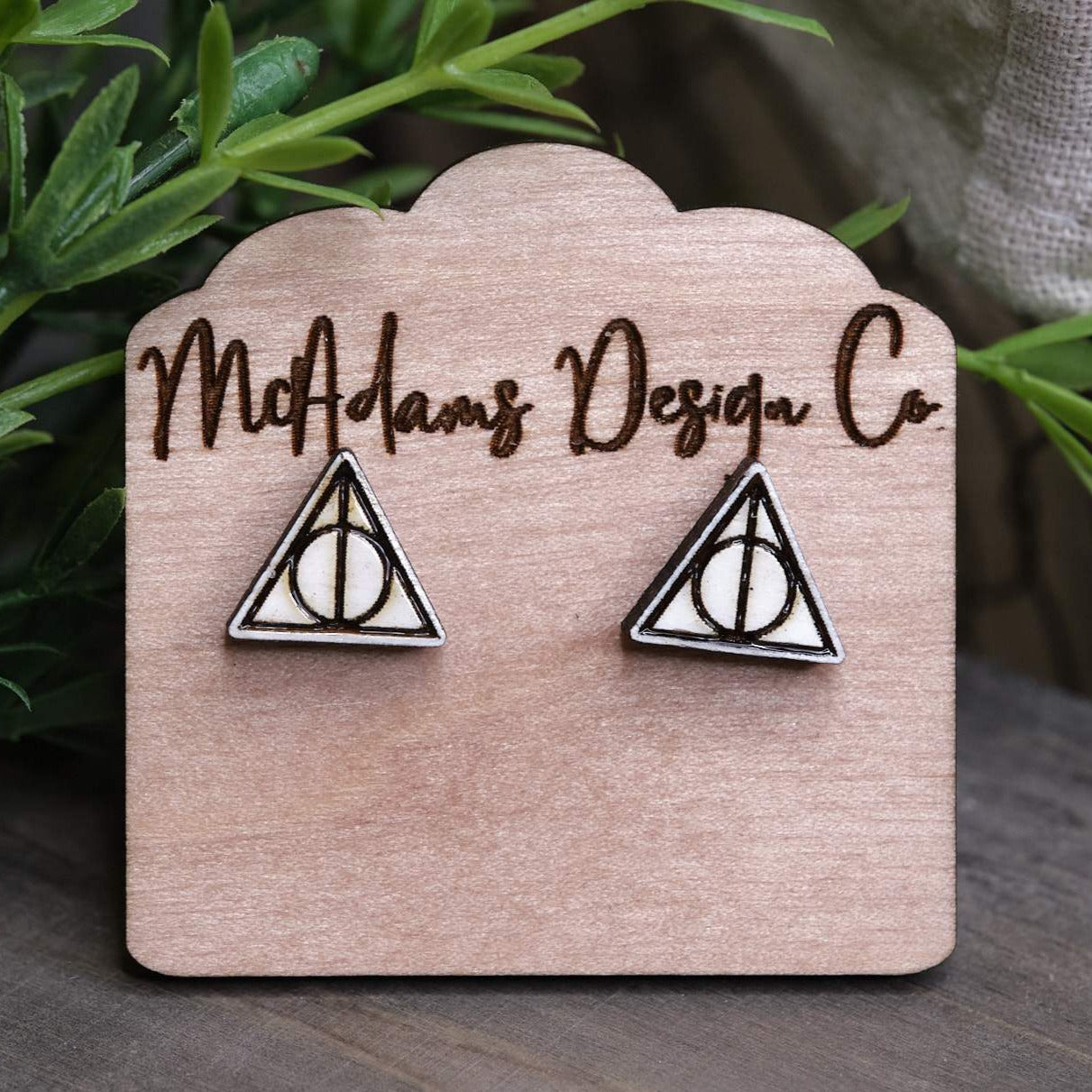The photograph showcases a sign that appears to be made from a material resembling wood, although its exact composition is unclear. The sign features a square shape with rounded edges, culminating in a distinctive, cloud-like curved top. The surface of the sign is light brown in color and prominently displays the inscription "McAdams Design Co." in a dark, cursive handwritten font. Below the text are two identical, equilateral triangle symbols, each with a black border. These triangles are segmented, containing an inner outline of another triangle bisected by a line, with a circle at the center. The triangles are not perfectly horizontal but rather slightly tilted. This sign is placed on a dark brown or gray table, and in the background, there is what appears to be an artificial plastic plant, recognizable by its green leaves visible at the top left of the image.